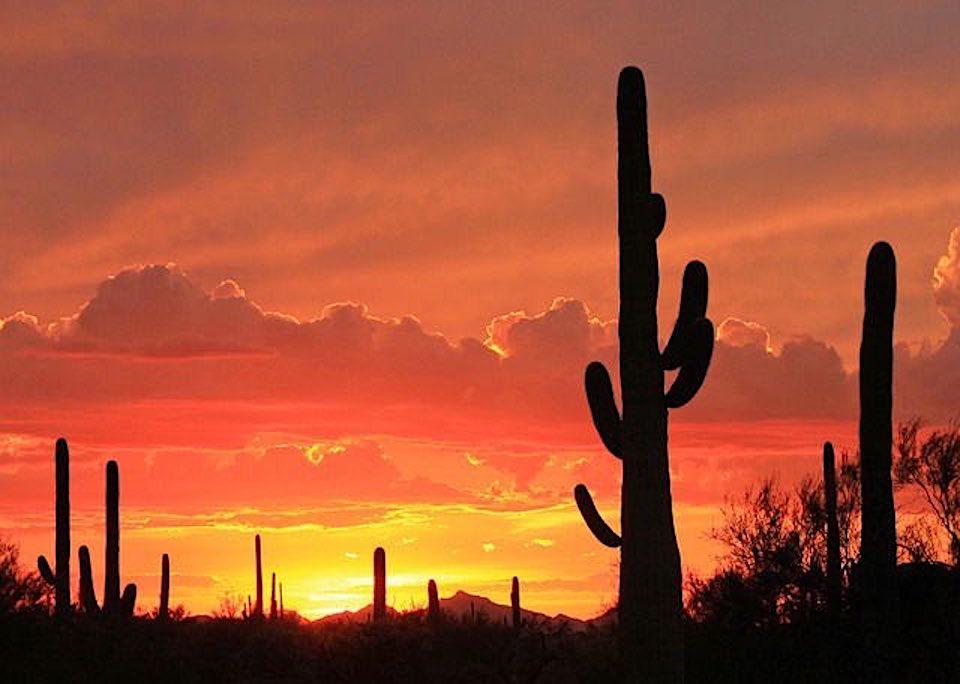This photograph captures a dramatic desert landscape at sunset, viewed from a low perspective. The sky is illuminated with deep hues of red, pink, and hints of purple, creating a strikingly vivid backdrop. The intense colors blend into bright yellows just above the horizon, where fluffy clouds, lit orange by the sun's low angle, scatter across the scene. In the foreground, the silhouette of a prominent Schrader cactus stands slightly to the right of the center, with two arms stretching out on either side. The cactus is surrounded by the shadowed outlines of additional cacti and some brush. Further back, a line of mountains traces the horizon, adding depth to the image. The sun, partially visible just above the mountains, casts long shadows and enhances the dramatic silhouettes of the desert flora, emphasizing their tall, imposing forms. This composition beautifully captures the serene yet rugged essence of a desert sunset.